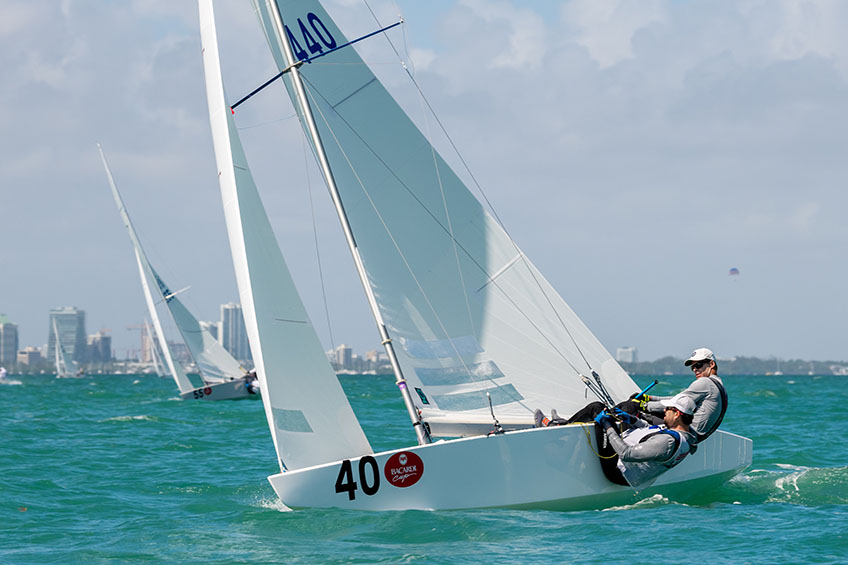In this detailed full-color photograph taken outdoors during the daytime using natural light, the focus is on a dynamic sailboat race set against an overcast sky with large clouds. Central in the image is a white sailboat, prominently marked with the blue number '440' on its sail and the black number '40' on its hull. The boat, appearing to tilt dramatically to the left, is manned by two men, both wearing gray shirts, white hats, and life jackets, who are leaning back so far it looks like they might fall into the water. They seem to be connected to the mast with harnesses and wires, counterbalancing against strong winds. The water below them has a greenish tint and appears slightly rough with some waves. In the left background of the image, another sailboat with the black number '55' on it can be seen, also engaged in the race. Farther back, the silhouette of a cityscape with tall buildings and skyscrapers is visible, providing an urban backdrop to this lively and detailed scene.